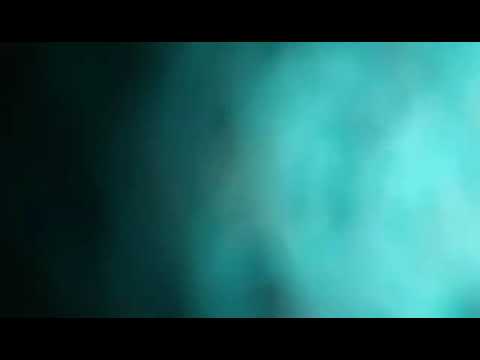The image is a roughly square photograph slightly wider than it is tall, with the top and bottom 10-15% blackened out in a letterbox fashion, reminiscent of widescreen movie frames. The central portion of the image features a gradient background pattern that transitions from light teal on the right to a deep black on the far left, mirroring the effect of descending into the depths of the ocean. This gradient is textured with wavy effects, creating the illusion of rippling water, adding dimension to the color shifts. The right side of the image is illuminated with a faint greenish light that intensifies in a wavy, smoky pattern towards the center, almost forming a nebulous, ghost-like face with eyes and a screaming mouth. The left side becomes progressively darker and less defined, as the greenish fog dissipates into deeper hues. Despite its textured appearance, the image is fairly basic and minimalistic, marked by compression artifacts and a soft, blurry gradient that enhances the ghostly and fluid nature of the scene.